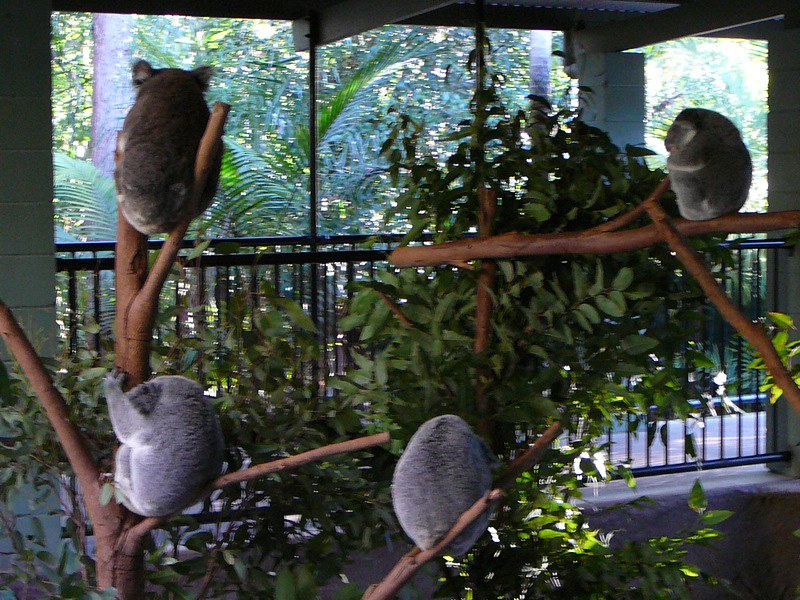In this detailed photograph, we see a group of plush, gray koalas ranging from grayish-brown to a lighter dusty gray, perched serenely on branches. These branches appear to be part of a carefully constructed display, suggesting a zoo enclosure. The koalas are seen clinging to these branches and munching on eucalyptus leaves, their fluffy forms facing away from the camera. 

The setting is an enclosed porch-like structure, complete with large screened windows that allow views of the lush, tropical foliage outside. The enclosure has a metal-fenced walkway for visitors to view the animals. The architecture features an overhanging roof that provides shade, reminiscent of Australian designs, reinforcing the impression that this could be a display mimicking an Australian habitat.

The environment is vibrant with greenery, and sun filters through, casting bright light on the scene. One koala is noticeably more visible from a side angle, with its head resting on its chest and front paws wrapped around a branch, resembling a big, round lump. This image captures the serene beauty and natural behavior of the koalas in a setting meticulously designed for their comfort and the viewer's enjoyment.